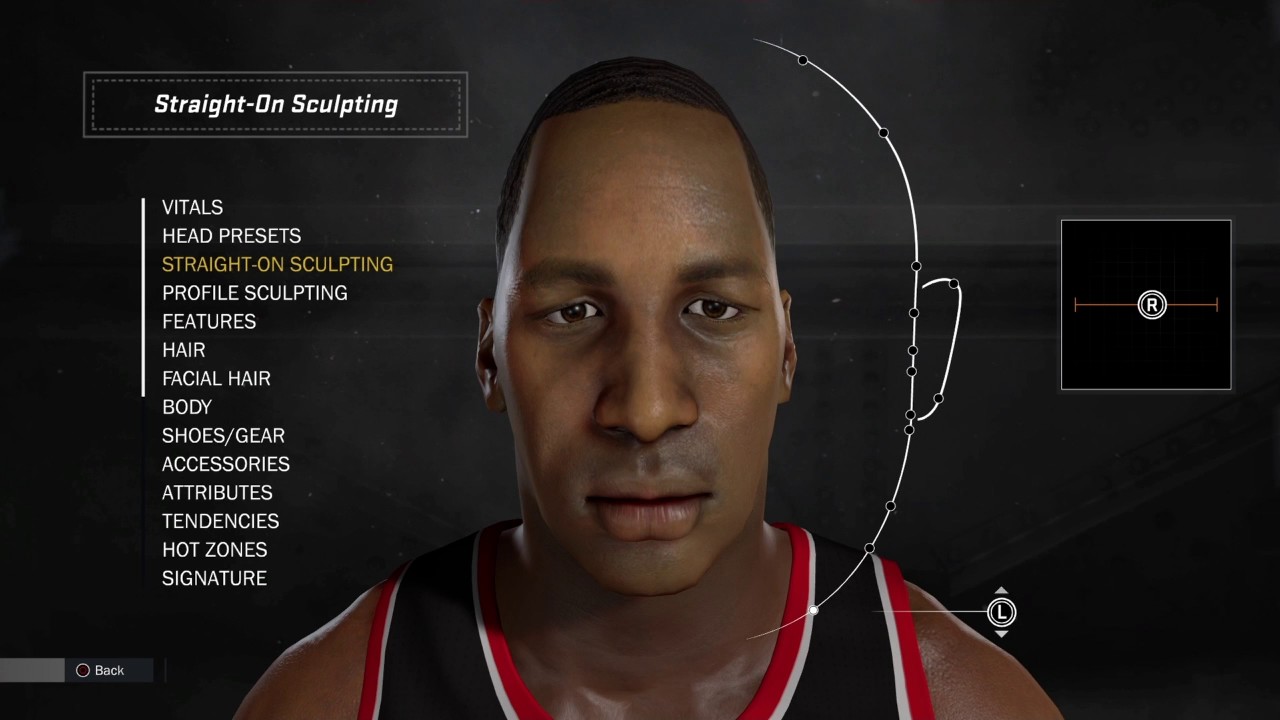A game player is meticulously designing a custom player in a popular basketball video game, likely from the NBA 2K series. The editing screen is focused on "Straight On Sculpting," as indicated by a label in the top left corner. The customizable character is an African American male with an elongated head, giving him a slightly exaggerated, almost cone-like appearance. His attire includes a black jersey with red trim. The robust customization interface offers numerous modification options, such as vitals, head presets, straight on sculpting (currently in use), profile sculpting, features, hair, facial hair, body, shoes, accessories, attributes, tendencies, hot zones, and signature moves. An interactive guide is visible on the screen, assisting the player in adjusting specific facial features like spacing and ear positioning."